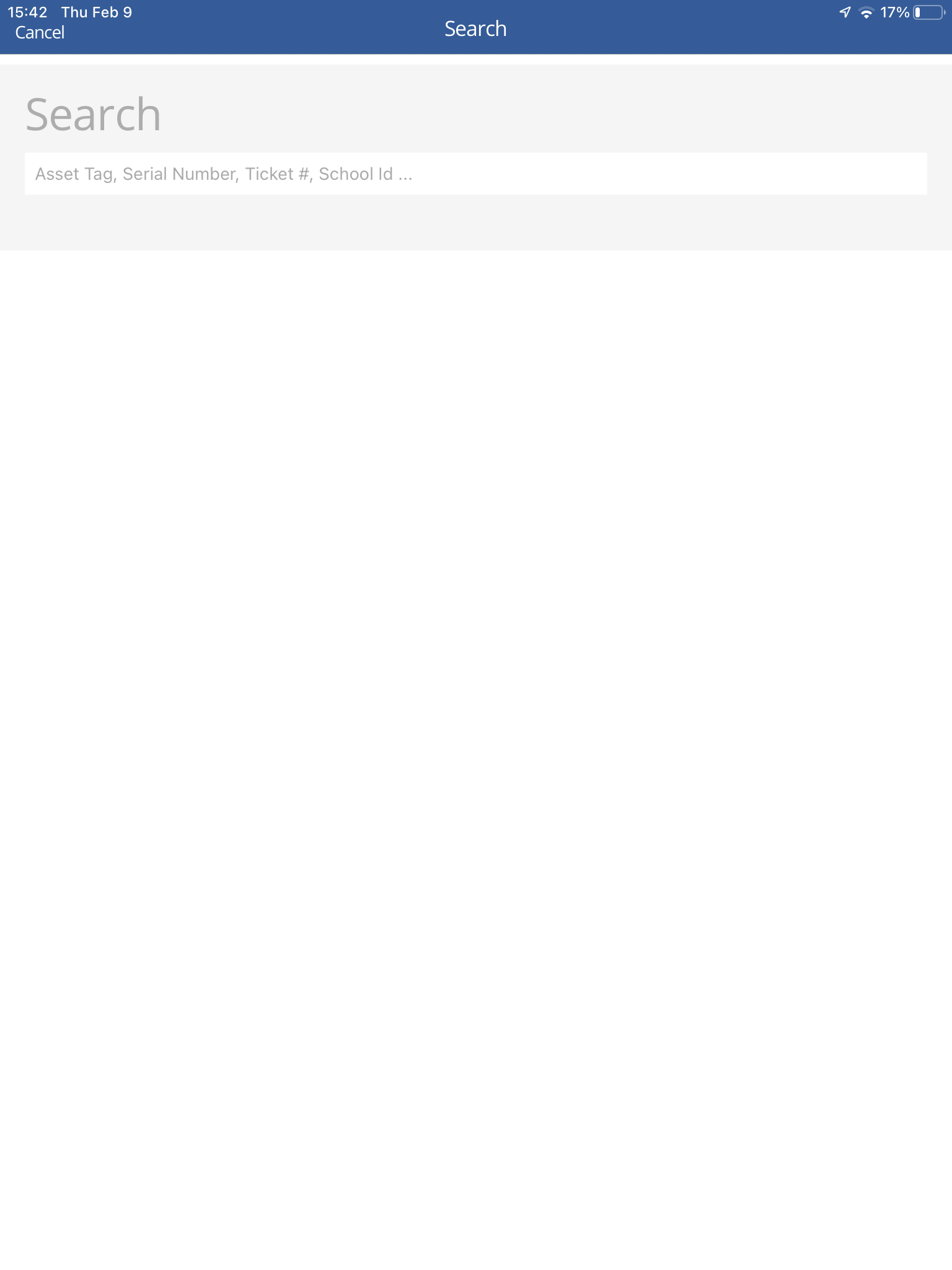This is a screenshot displaying a section of an application on a mobile or tablet device. At the top, there is a dark blue header bar, characterized by its short rectangular shape. In the top left corner, the time is shown as 15:42. Adjacent to the time is the date, written as THU, FEB 9. Slightly to the left, in white letters, is the word 'CANCEL'.

Centrally positioned and slightly lower from the top edge of the header, the word 'SEARCH' is prominently displayed in white. On the top right, there are four icons arranged from left to right: an outline of an arrow pointing up and to the right, a Wi-Fi symbol with three bars (two of which are filled white, and the top one is gray), a numeric indicator showing '17%', and a horizontal battery icon with a white bar indicating it is 17% charged.

Below this header, a thin white line separates it from the body of the page. The body begins with another header that has a light gray background. At the top left of this lighter header, the word 'SEARCH' appears again in large, dark gray, sans-serif text.

Beneath this, there is a white search bar nearly spanning the entire width of the gray header. Inside the search bar, light gray placeholder text reads 'ASSET TAG, SERIAL NUMBER, TICKET #, SCHOOL ID, ...', with each term separated by a comma. 'SERIAL NUMBER' includes the word 'NUMBER,' and 'TICKET #' uses a pound symbol in place of the word 'NUMBER'.

The remainder of the screen beneath the gray header is a large, white area.